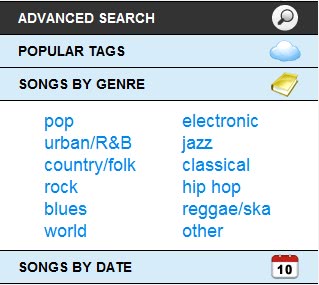Screenshot of a music app interface displaying a categorized list of songs. The layout is divided into four main sections. At the top is the "Advanced Search" section, indicated by a magnifying glass icon. This section likely features a button that, when pressed, brings up a search bar for more specific queries.

Directly below that is the "Popular Tags" section, marked by a cloud icon. This section isn't expanded but serves as a gateway for users to explore commonly used music tags.

The third and prominently detailed section is "Songs by Genre," identified by a book icon. This section is expanded to reveal a comprehensive list of music genres. The genres are displayed in blue text and organized into two columns, enhancing readability. The genres listed include: 

- Pop
- Urban/R&B
- Country/Folk
- Rock
- Blues
- World
- Electronic
- Jazz
- Classical
- Hip-Hop
- Reggae/Ska
- Other 

Finally, the fourth section is "Songs by Date," easily recognizable by its calendar icon. This section is not expanded, indicating it may contain a sortable list of songs based on their release dates when accessed.

Overall, the image offers a well-structured menu for navigating through a diverse range of music options within the app.